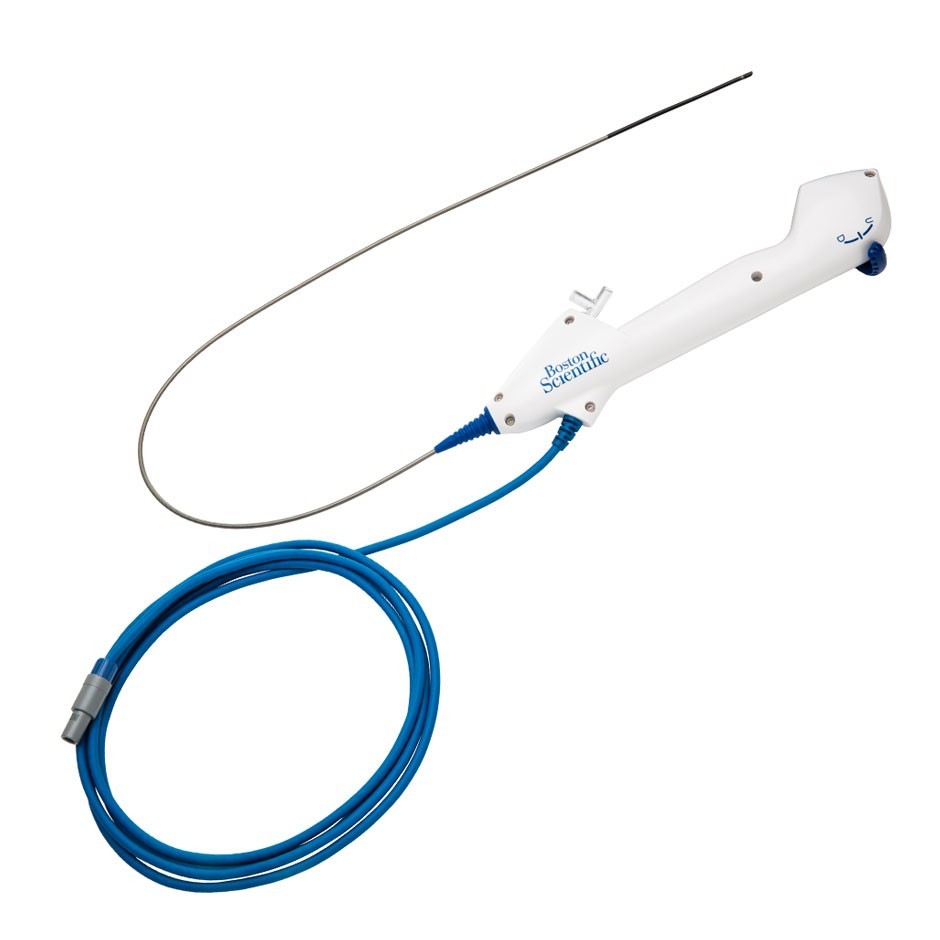The image showcases a medical device produced by Boston Scientific, prominently featuring their name in blue lettering on a sleek, white handle. The device resembles an electric toothbrush but is likely intended for clinical use. Emerging from the device are two distinct wires: one is a long, blue cord that loops neatly, likely for connecting to another machine or a receiver, while the other wire extends upward and could be a receiver or sensor wire. The handle itself incorporates a gray tip and includes a knob at the bottom that can be flicked on and off. Additionally, there's a button near the upper section, presumably to activate the device. The entire setup is set against a clean, white background, enhancing its clinical appearance and suggesting its use in medical settings, potentially for respiratory or other hospital-related applications.